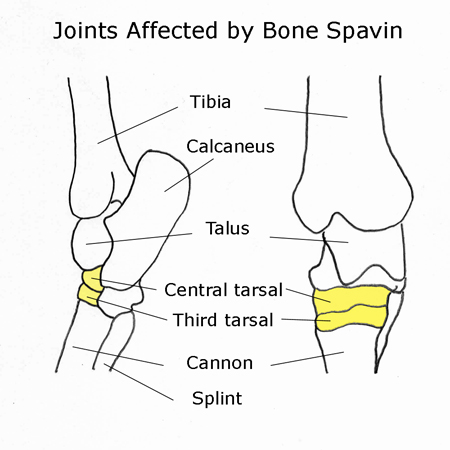The image is an anatomical poster titled "Joints Affected by Bone Spavin," illustrating the knee area of the leg. It primarily features black-and-white diagrams with some parts highlighted in yellow. The diagram includes detailed labels for various bones and joints: the tibia, calcaneus, talus, central tarsal, third tarsal, canon, and splint. The poster showcases these areas from multiple angles, with a frontal view on the left side and a rear view on the right side. The notable highlights in yellow on the central tarsal and third tarsal indicate areas of particular interest or affliction, possibly due to bone spavin. This educational illustration is likely used in a classroom setting to explain the anatomical structure and joint locations in the leg.